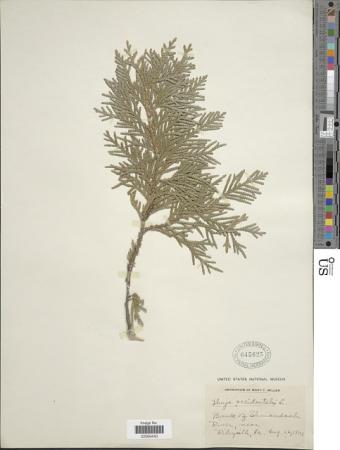In this photograph, a greeting card's back is depicted, shot from a distance, not up close. The card has a cream-colored background with a tree motif intricately etched, potentially in gold leaf, highlighting a skinny, prominent, vertical tree with numerous branches. A green leaf, compared by some to an Arborvitae or cedar sprig, is also imprinted on the card, appearing from the tree's branches. The leaf has been described as somewhat unattractive in hue. At the bottom of the card, a white barcode and some small, hard-to-read print are visible. Additionally, on the top right, there's a color palette or grid, likely from a computer program, suggesting that the card might be in the process of being modified digitally. There's also some handwritten text, possibly part of the card's design. This photograph seems to capture the card as part of a design or proofing process, indicated by the presence of editing software elements.